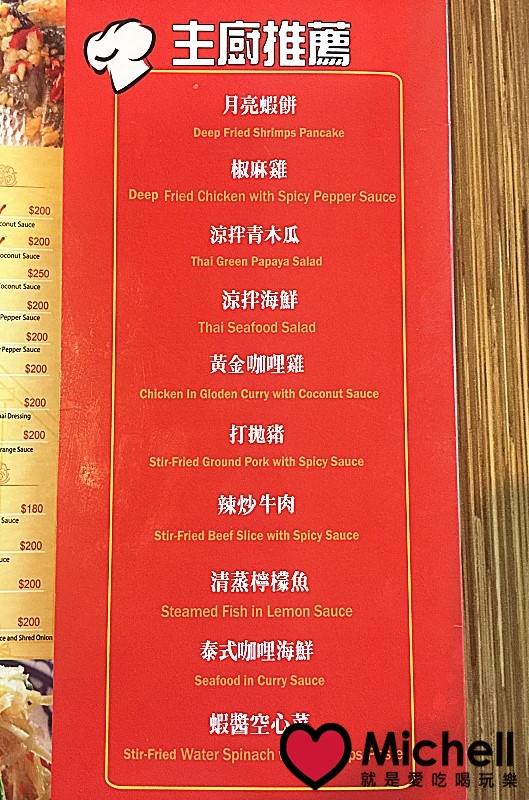The image depicts a red menu board adorned with Chinese writing at the top, alongside a whimsical white cartoon drawing of a chef's hat situated to the immediate left of the text. Centrally positioned on the board is a rectangular, golden-bordered section containing the names of various dishes, presented both in Chinese characters and English text. The English names are rendered in a brown or deep gold hue. The listed dishes are:

1. Deep Fried Shrimp Pancake
2. Deep Fried Chicken with Spicy Pepper Sauce
3. Thai Green Papaya Salad
4. Thai Seafood Salad
5. Chicken and Gold Curry with Coconut Sauce
6. Stir Fried Ground Pork with Spicy Sauce
7. Stir Fried Beef Slice with Spicy Sauce
8. Steamed Fish in Lemon Sauce
9. Seafood in Curry Sauce
10. Stir Fried Water Spinach (the rest of this menu item is obscured by a red heart watermark with a black border and the text "Michelle").

Flanking the menu board to the right is a wall featuring dried bamboo, adding a rustic element to the scene. To the left, another section of the menu set against a gold background displays additional pricing information for various items.